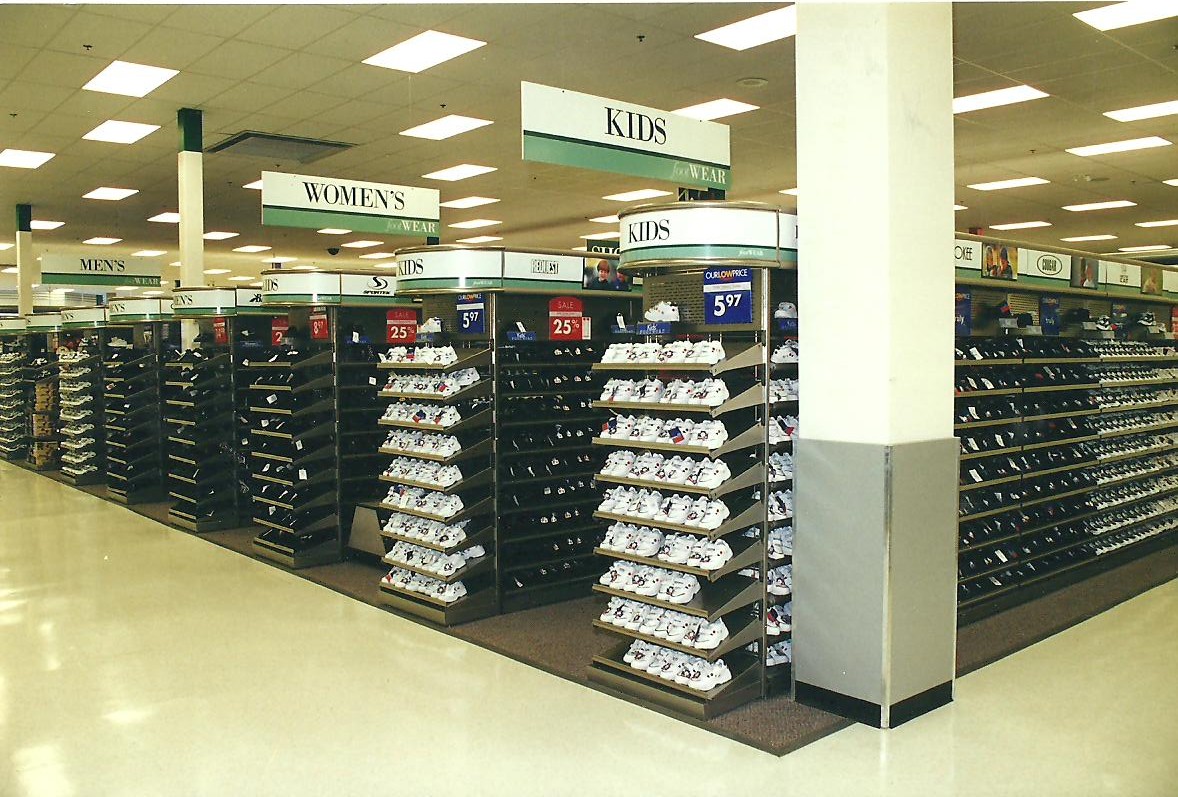This photograph captures the interior of a bright, well-lit shoe store or shoe section within a department store. The floor is a shiny white-beige linoleum in the walkways, transitioning to carpeted areas where the shoes are displayed. Prominent in the foreground is a large white pillar with a silver box around it and a black stripe. The store features tall, organized shelving units running diagonally, approximately six feet high, displaying various rows of shoes. The first section encountered is the kid's section, prominently showcasing rows of white tennis shoes priced at $5.97 on the end caps. Signs in the background identify sections clearly: "Women's" in black lettering on a white sign above a green "Footwear" label, and "Men's" further behind. The ceiling consists of rectangular panels with evenly spaced artificial lighting, contributing to the store’s bright ambiance. Notably, the image depicts orderly, clean rows of shoes with no people present.